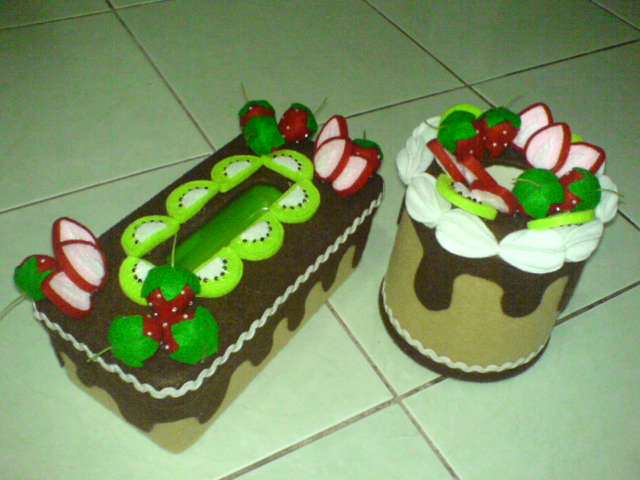The photograph showcases two intricately decorated felting material containers designed to resemble delectable desserts. Positioned on a cream-colored tile floor with beige grout, the meticulously crafted containers bring a vibrant, whimsical charm to the setting.

On the left, a rectangular box mimics a long tissue box, featuring a beige base with dark brown chocolate-like drips along the edges. Topping the faux cake are white rickrack icing and an array of green kiwi slices arranged around the center slit. At either end, whole strawberries with green leaves and sliced radishes add bursts of realistic color.

To the right, a cylindrical container, resembling a large cupcake or a toilet paper holder, mirrors the chocolatey, beige design. Its detailed decorations include a bottom layer of dark brown, a midsection of realistic white cream, and a crowning assembly of strawberries, kiwi, and radish slices. Puffy white icing details further enhance its cake-like appearance.

Both containers echo a unified pastry motif, skillfully adorned with felt fabric to imitate the textures and vibrant aesthetics of real desserts, creating an endearing, surreal visual.